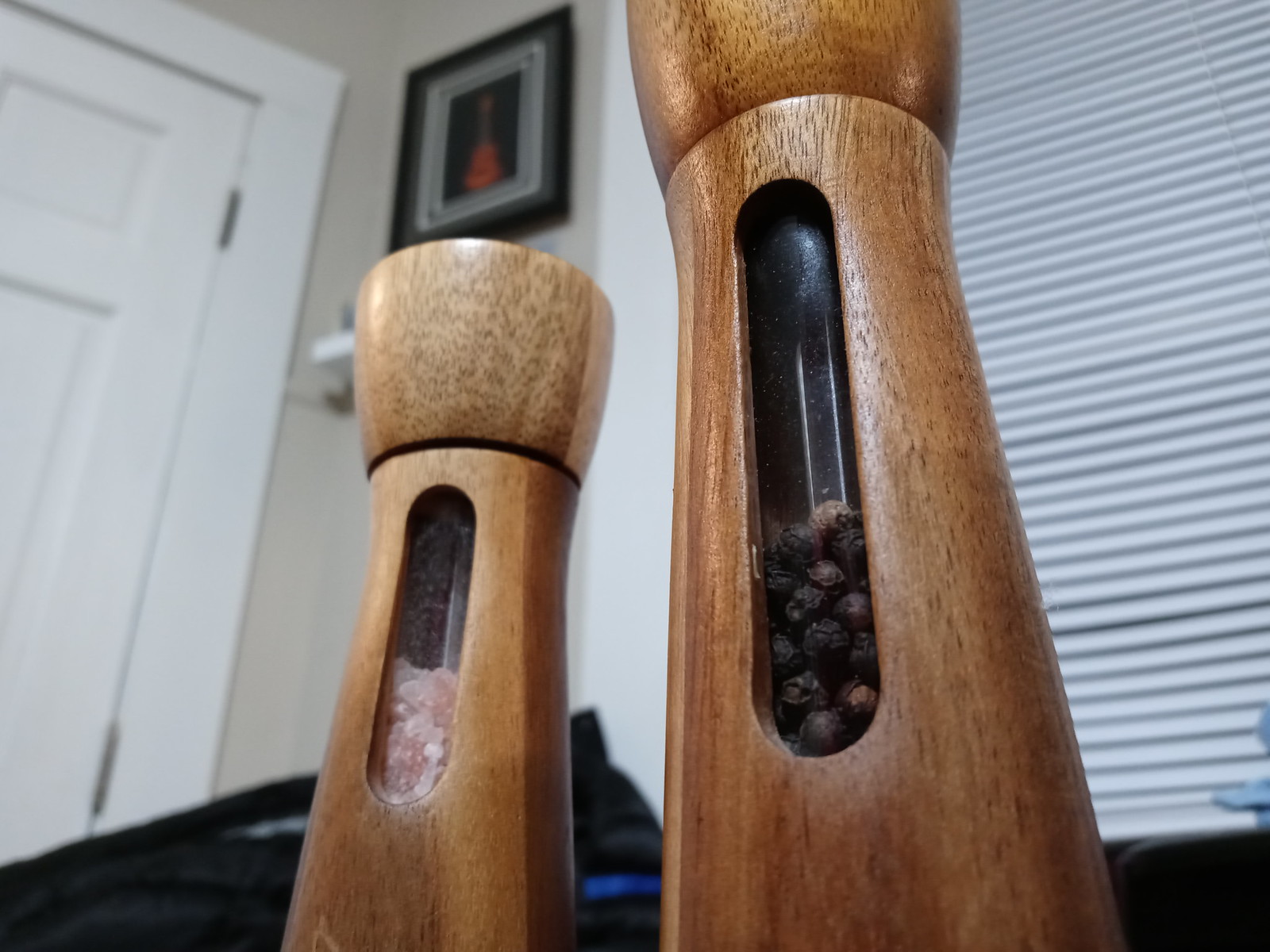In the foreground of this detailed image, there are two large wooden salt and pepper grinders with rounded tops designed to twist for grinding. The salt grinder is filled about a quarter of the way with what appears to be pink Himalayan salt, and the pepper grinder is filled about a quarter and a half with black peppercorns, which are clearly visible through the small windows on the front of each grinder. The setting seems to be a kitchen or dining room in someone's house. 

In the background, a light-colored wall features a black-framed photo hanging above a small shelf. To the left of the wall, there's a white door with a matching frame. A window on the wall has closed horizontal mini blinds. Additionally, there seems to be a black cloth or coat partially visible and a light blue pitcher or bowl. The overall scene is framed in such a way that it is unclear whether the grinders are placed on a table or another surface.